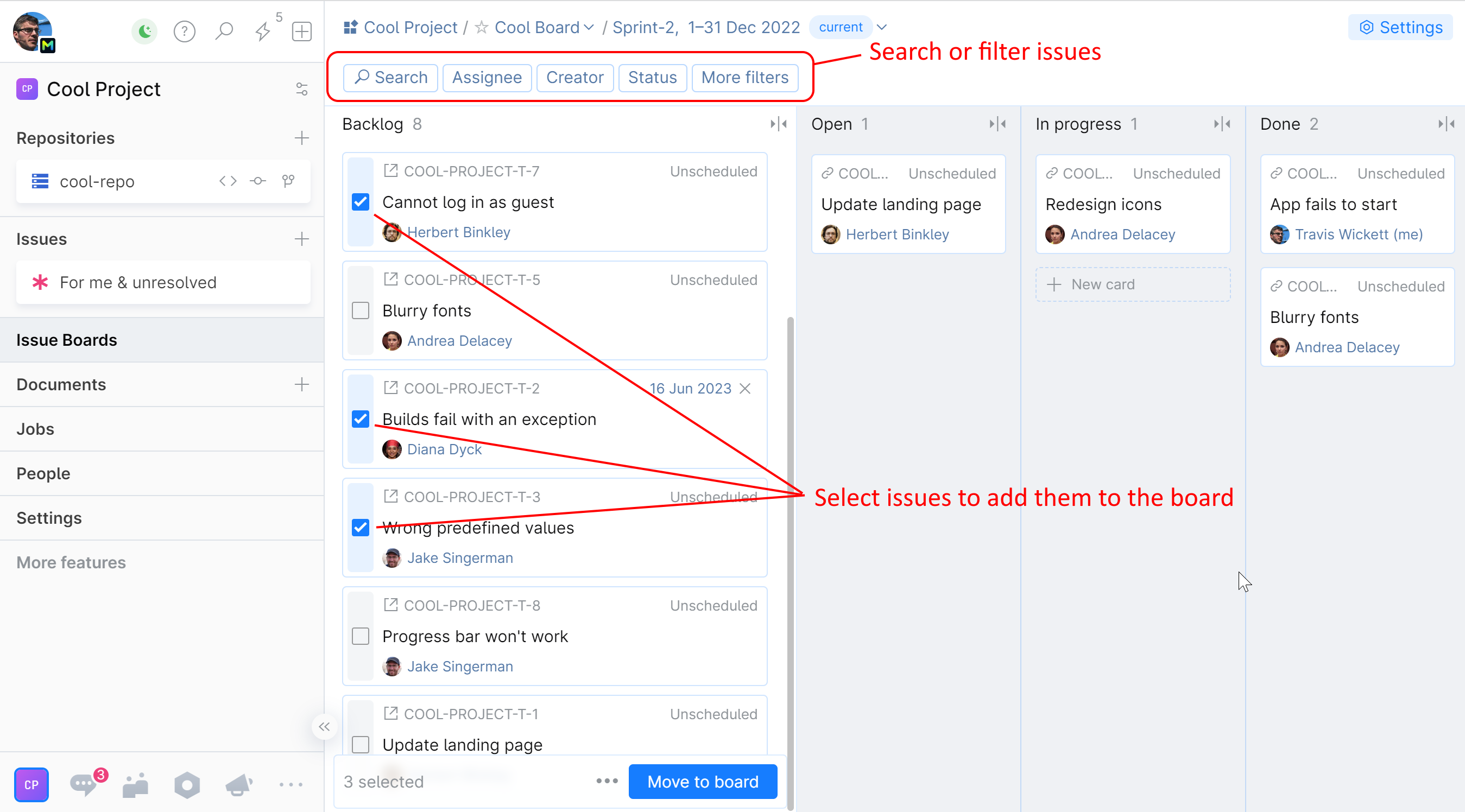The image depicts a detailed interface for a project management system, likely used in a school or educational environment. In the upper left-hand corner, there is a small portrait of an older man. Directly beneath this image is a purple box labeled "Cool Project," followed by several navigational options: "Repositories," "Issues," and "Issue Boards." A red asterisk next to "Issues" indicates one unresolved issue.

Under the "Issue Boards" section, the following options are listed: "Documents," "Jobs," "People," "Settings," and "More Features."

On the second screen, a prominent red rectangular box at the top contains search and filtering options: "Search," "Assignee," "Creator," "Status," and "More Filters." Below this, a directive states, "Search or filter issues," illustrated by a connecting line from the red box.

The backlog list shows several issues:
1. "Cannot log in as a guest" - Marked with a blue check and linked to "Select issues to add them to the board."
2. "Blurry fonts" - Unchecked.
3. "Builds fail with an exception" - Checked with a red line leading to the issue selection board.
4. "Wrong predefined values" - Also checked with a red line leading to the issue selection board.
5. "Progress bar won't work" - Listed without additional annotations.
6. "Update landing page" - Initially to be moved to the board but later not included in the tasks.

A blue button at the bottom labeled "Move to Board" is used to finalize issue selection. The update confirms that "Update landing page" was deselected.

In the third column, issues labeled "Apps fail to start" and "Blurry fonts" appear again, suggesting they are the rejected items. The final item in the column is "Redesign icons," indicating ongoing or completed tasks.

This organized setup allows users to efficiently manage and track project issues and progress, with specific attention to unresolved and pending tasks.